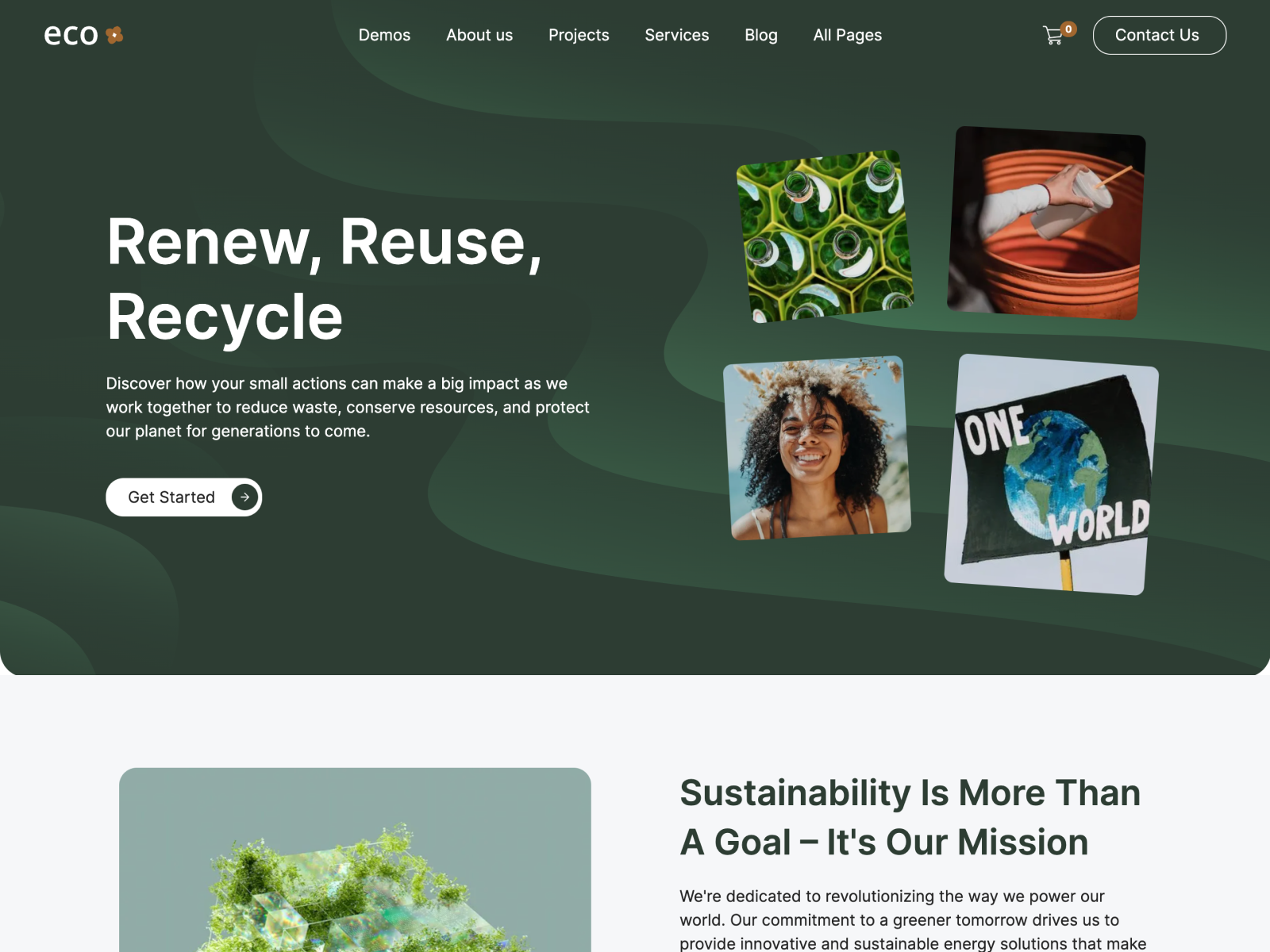The image is a detailed screenshot of a website belonging to a company called Eco. The website header features tabs for Demos, About Us, Projects, Services, Blog, and All Pages. In the top left corner, the Eco logo is displayed, and in the top right corner, there is a shopping cart icon with zero items in it, alongside a "Contact Us" link. 

The website's design prominently features a dual-colored background, with the upper section in green and the lower section in white. On the green section, the message "Renew, Reuse, Recycle" is highlighted, emphasizing the website's ecological focus. Below this, a paragraph elaborates, "Discover how your small actions can make a big impact as we work together to reduce waste, conserve resources, and protect our planet for generations to come." 

A "Get Started" button is situated to the right of this text, accompanied by instructions on recycling practices, such as how to dispose of glass and plastic bottles. There are multiple images integrated into the layout, including one of a smiling woman, vibrant and sunny, and another showing someone properly discarding items into a recycling bin. A notable banner reads "One World," promoting the idea of global unity in sustainability efforts. 

Further down, another prominent message states, "Sustainability is more than a goal; it's our mission. Our commitment to a greener tomorrow drives us to provide innovative and sustainable energy solutions." Additional images show various eco-friendly actions, such as a collection of glass bottles, reinforcing the site’s dedication to environmental conservation and sustainable living.